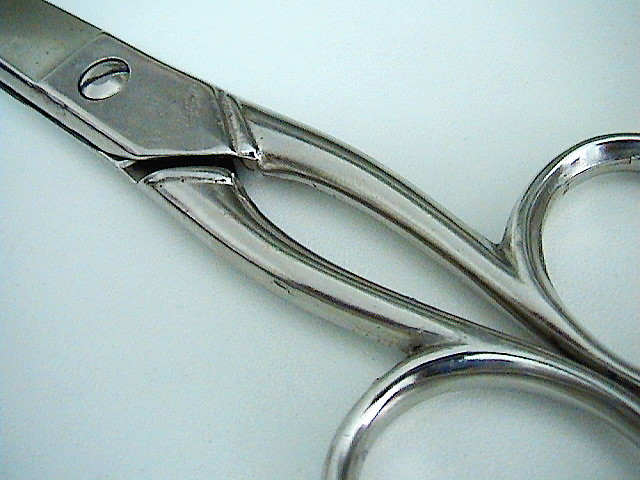This is a close-up photograph of an aged pair of silver metal scissors, likely chrome-finished, against a light off-white or slightly grayish background that darkens toward the lower right corner. The image captures only the top part of the round handles and the upper section of the blades, which are held together by a single screw. The scissors appear slightly old with visible markings, scratches, and some rust. The metal material of the scissors catches the light, casting a distinct shadow to the bottom right of the scene.